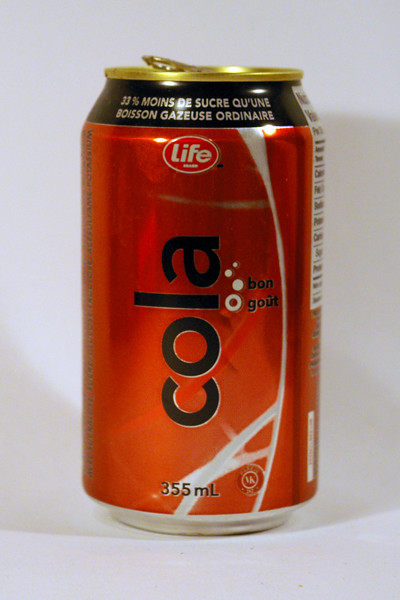The image depicts a sophisticated photographic diorama showcasing an aluminum can of French cola, primarily characterized by its red background and tasteful accents in white. The rectangular can features black text that spells "cola" in lowercase letters, prominently positioning the beverage name over its brand. Above a gold lip lies a black band adorned with French text, which sits beneath the signature gold top tab. This subtle yet refined can, embossed with a circular "Life" brand logo in bold white text within a red oval, appears almost generic, as the cola itself takes precedence. Further detailing includes a distinctive white streak starting wider at the top and tapering down as it wraps around the can, alongside an additional thick white line originating from the middle and running upward. Notably, the bottom band of the can is silver, and the label also specifies a volume of 355 milliliters. Additionally, a glimpse of the nutritional facts is visible on the right edge of the can.